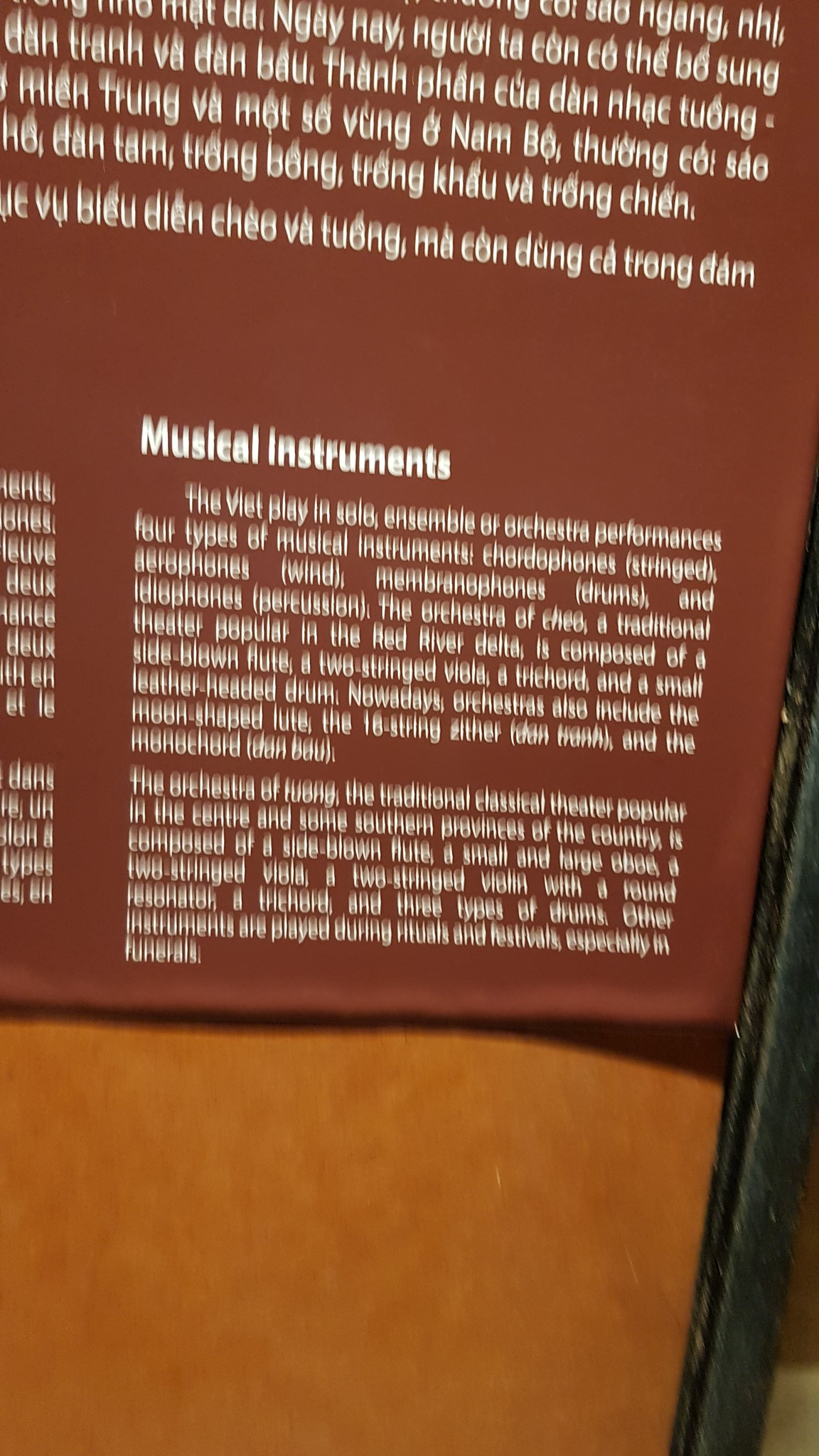The image showcases a sign mounted next to a wall. The sign, colored in a dark red-brown hue, features a block of Vietnamese text at the top. Below the text, there are illustrations of various musical instruments. Beneath these illustrations, two blocks of English text are arranged. On the left side, partially cropped out of the image, are two more blocks of text. The wall behind the sign is a lighter brown shade, creating a contrast with the sign. A black strip is visible on the right side of the image, extending vertically alongside the sign. Subtle shadows cast by the sign can be seen on the wall, adding depth to the scene.